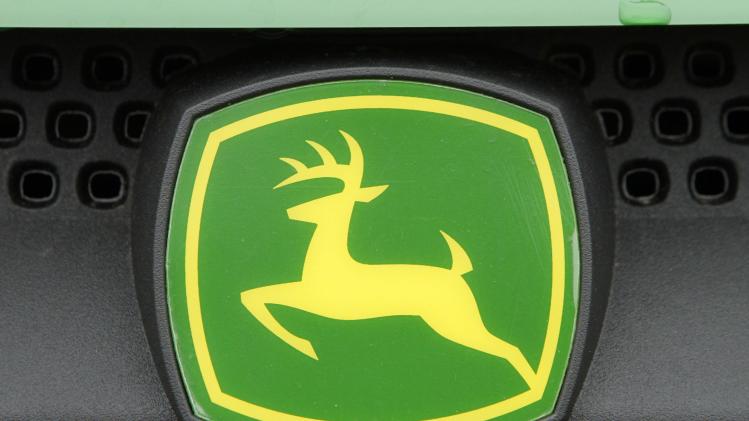The image is a close-up of the John Deere logo prominently displayed on a piece of machinery, likely part of a tractor or other farm vehicle. The John Deere symbol, featuring a yellow deer in mid-leap with its front legs off the ground, is set against a bright green background and surrounded by a yellow border. The logo, characterized by its square shape with convex sides, is mounted on a grey base with various holes and protruding rods, suggesting it could be part of an air intake system or another functional component. The top of the logo features an additional line border that is not part of the mounting. The surrounding area of the image is mostly black, possibly indicating it is made of plastic or another darker material. The detailed depiction of the deer includes visible antlers, affirming its male identity.